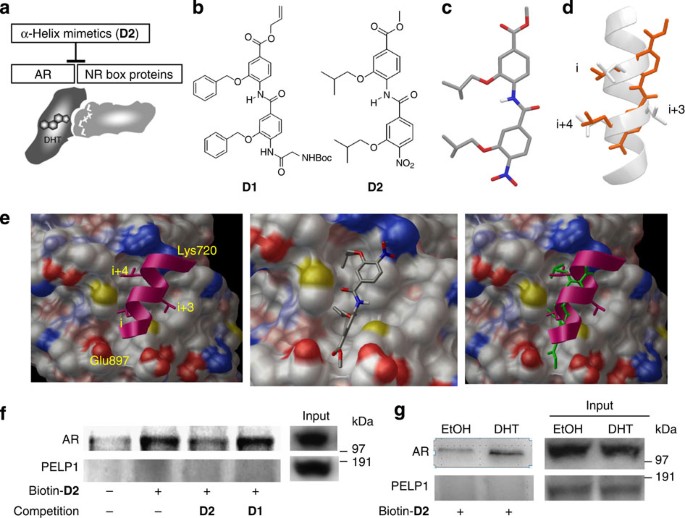The image resembles a detailed infographic often seen in a chemistry or biology textbook, featuring diagrams of DNA strands and various proteins. It has a white background, and the content is organized into sections labeled A through G. At the top, section A shows helix mimetics and ARNR box proteins, illustrated with gray masses containing protein structures. Sections B and C depict black-and-white diagrams of protein structures, with C introducing color; it shows hexagons connected by lines marked with O, OH, and N groups. Section D features a colored spiral helix structure with orange elements indicating protein interactions. Moving to the middle, the diagrams include gray, red, and blue balls representing digital illustrations of molecular structures against a white, blue, and yellow backdrop. The bottom section contains labeled boxes such as AR, PLP1, biotin D2, and competition, resembling x-ray images with gray and black stripes. Sections F and G display graphical readings or data likely related to the DNA strands and proteins, completing the intricate layout of biochemical information.